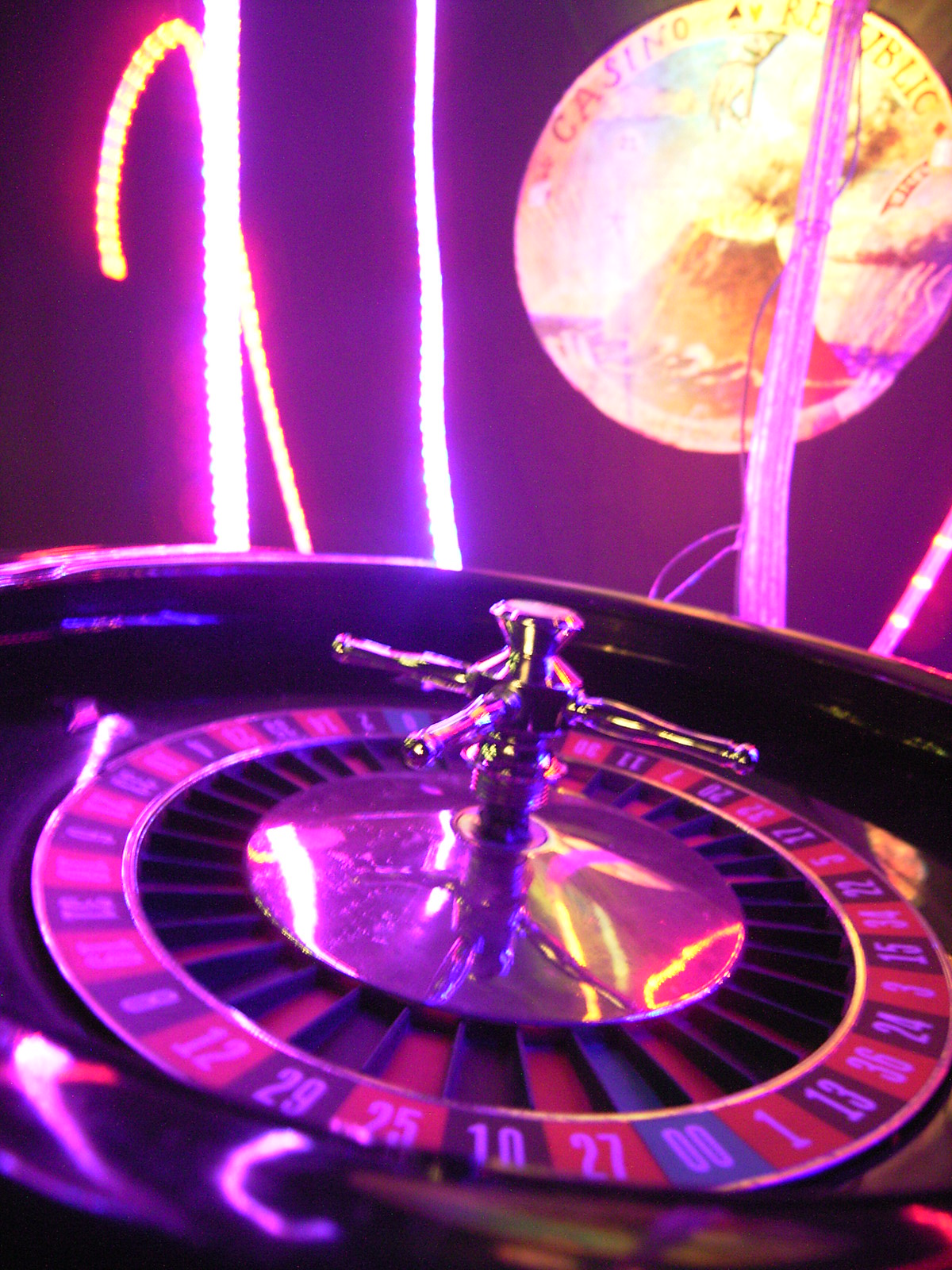The image showcases a blurry, out-of-focus photograph of a roulette table inside a casino. Dominating the shot is the roulette wheel at the center of a round table, featuring multiple numbers in white on alternating red and black squares with green for the zero and double zero. The wheel's inner mechanism appears to have a chrome finish, accented with what looks like gold handles. Behind the roulette table, the back wall is illuminated by haphazardly hanging LED string lights casting purple and pink hues, with one strip noticeably drooping. A backlit sign on the far wall reads "Casino Republic" and includes a hand-drawn depiction of a volcano erupting, infusing the scene with a vibrant, neon aesthetic.